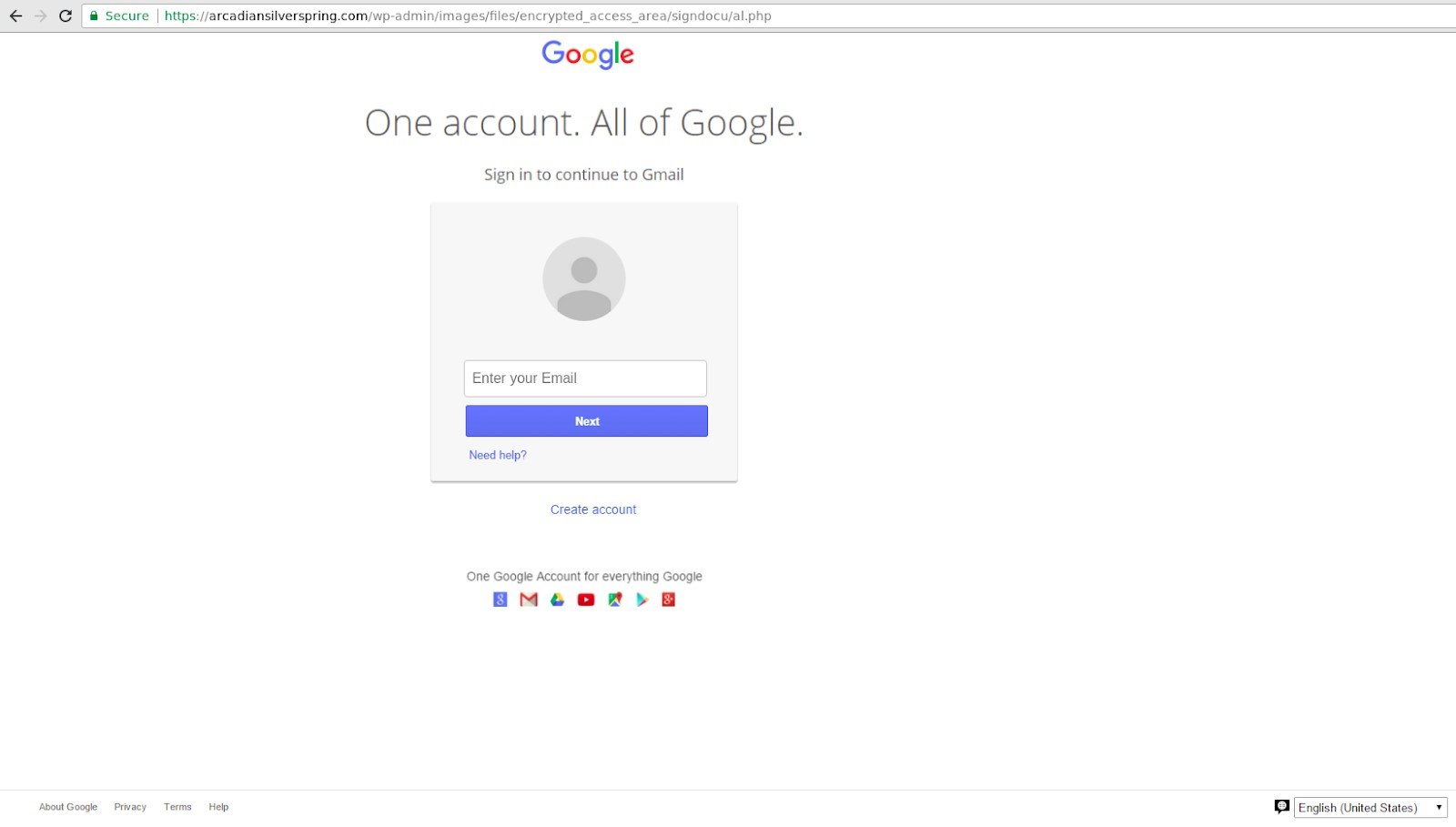The screenshot displays a secure desktop application interface, as indicated by the HTTPS prefix in the search bar. The URL reads: "arcadiansilverspring.com/wp-admin/images/files/encrypted_access_area/sign_docu/al.php." 

At the top of the interface, there is a prominent Google logo, followed by the text "One account. All of Google. Sign in to continue to Gmail." Below, there is a profile picture placeholder, alongside an input field labeled "Enter your email," with a blue "Next" button positioned underneath.

Further down, there are hyperlinks stating "Need help?" and "Create account." The phrase "One Google account for everything Google" is positioned below these links, accompanied by a collection of Google application icons, including Gmail, Google Drive, YouTube, and the Android app logo, among others.

In the bottom-right corner of the screen, the language setting is displayed as "English (United States)," with a dropdown menu. To the left, there is a series of small links labeled "About Google," "Privacy," "Terms," and "Help."